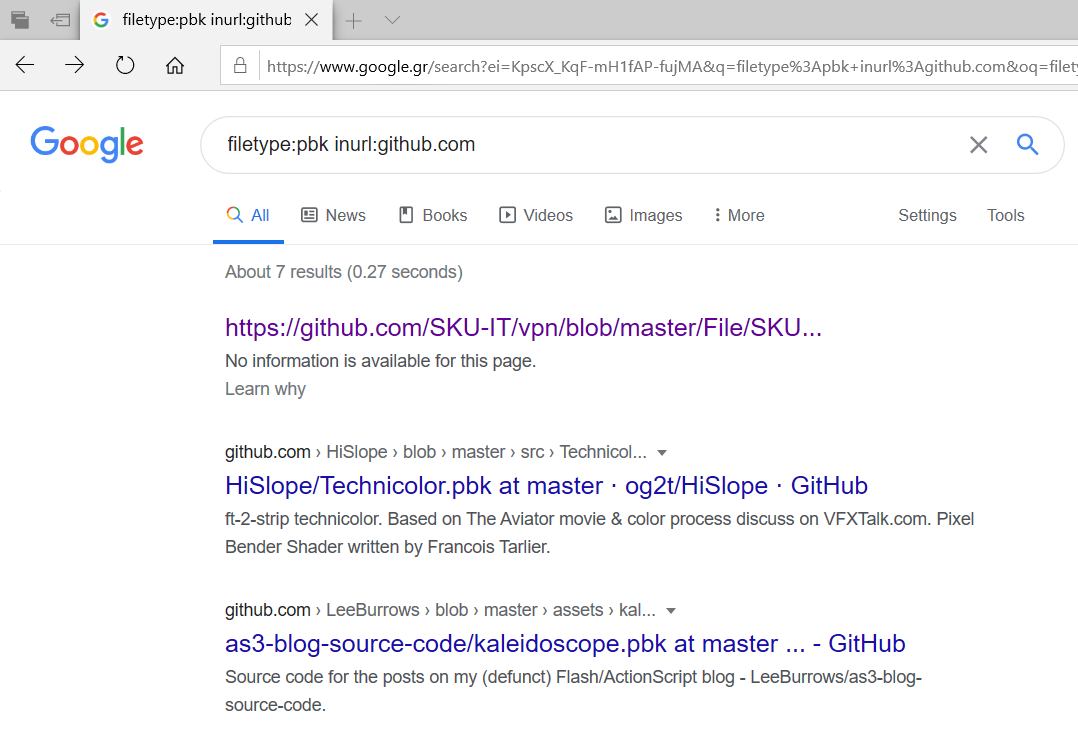**Detailed Caption:**

The image depicts a Google search results page with the following elements:

1. At the top of the screen, next to the Google logo, the search query reads: `filetype:pbk inurl:github`.

2. The Google search bar is prominently displayed, filled with the aforementioned query. The URL of the search results page begins with "google.com/search" followed by a string of alphanumeric characters.

3. The colorful Google logo is positioned to the left of the search bar. The logo consists of a blue "G", a red "o", a yellow "o", a blue "g", a green "l", and a red "e".

4. Below the search bar, there is a results summary stating that approximately seven results were found in 0.27 seconds.

5. The first search result is a clickable link to GitHub.com. The linked text reads "No information is available for this page."

6. Below the link, a smaller text shows the URL path as "GitHub.com -> highslope-technicolor.pbk at master.og2t highslope.github".

7. The second search result refers to another part of GitHub, specifically "AS3 blog source code/kaleidoscope.pbk at master.github".

8. This result is accompanied by a gray text description: "Source code for the posts on my Flash-ActionScript blog."